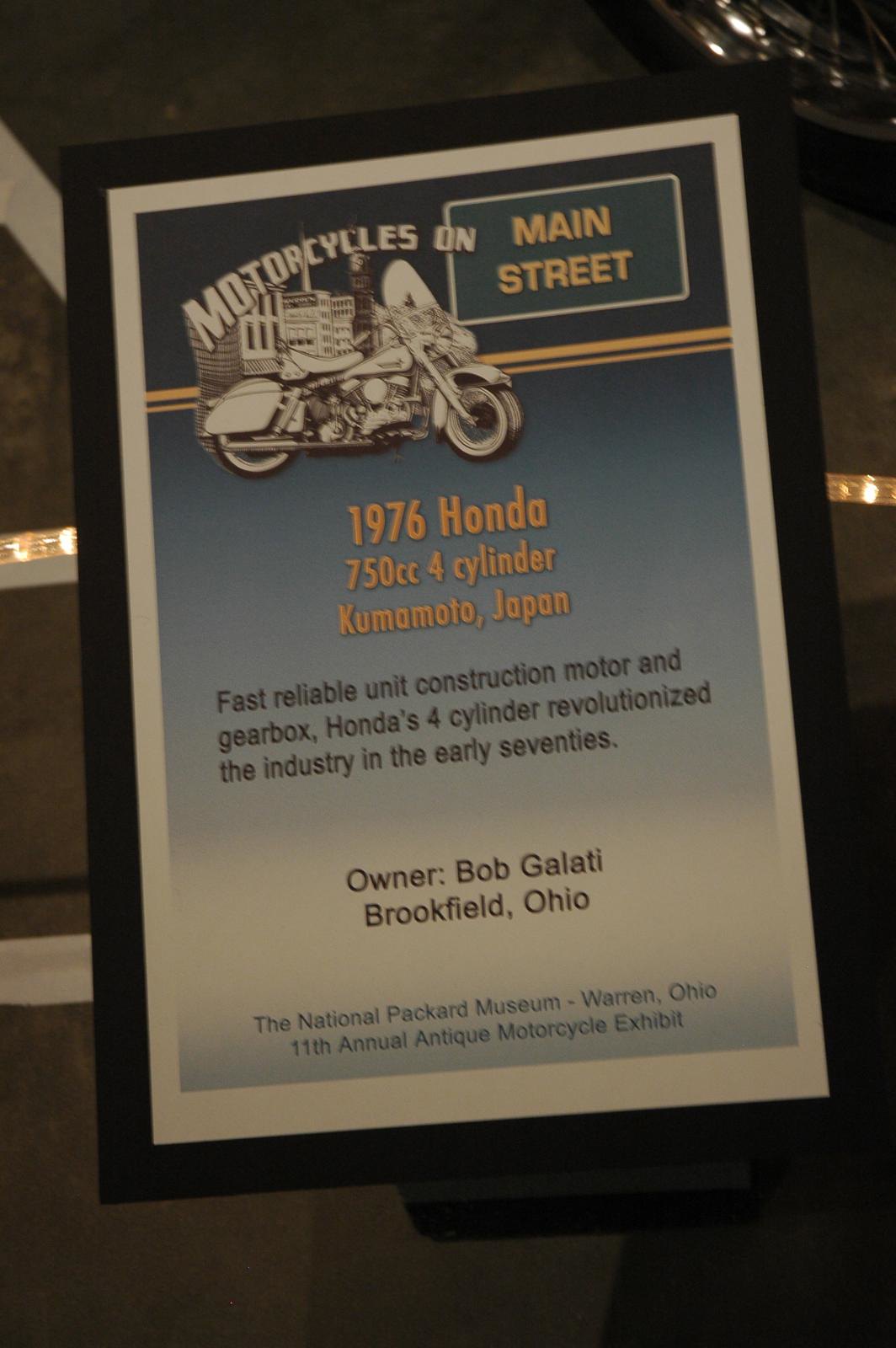This detailed photograph showcases a commemorative plaque likely situated in a museum or indoor exhibit, possibly within a parking garage. The plaque is designed with a white frame bordered by a black frame resting on a surface. At the top, in color, it prominently features the text "Motorcycles on Main Street" along with an illustration of a motorcycle set against a city skyline, depicted in a black and white sketch style with a red and yellow street sign reading "Main Street."

The center of the plaque captures attention with a detailed description in orangish-yellow text: "1976 Honda, 750cc, 4-cylinder, Kumamoto, Japan," followed by a smaller black text detailing the bike's attributes: "Fast, reliable unit, construction motor and gearbox. Honda's four-cylinder revolutionized the industry in the early 70s."

Beneath the technical description, the owner's name and location read "Owner Bob Galati, Brookfield, Ohio." The bottom of the plaque is marked with blue text indicating its exhibit: "The National Packard Museum, Warren, Ohio, 11th Annual Antique Motorcycle Exhibit." This plaque serves not only as an informative piece about the displayed motorcycle, a 1976 Honda 750cc four-cylinder, but also as a tribute to its historical significance and its owner.